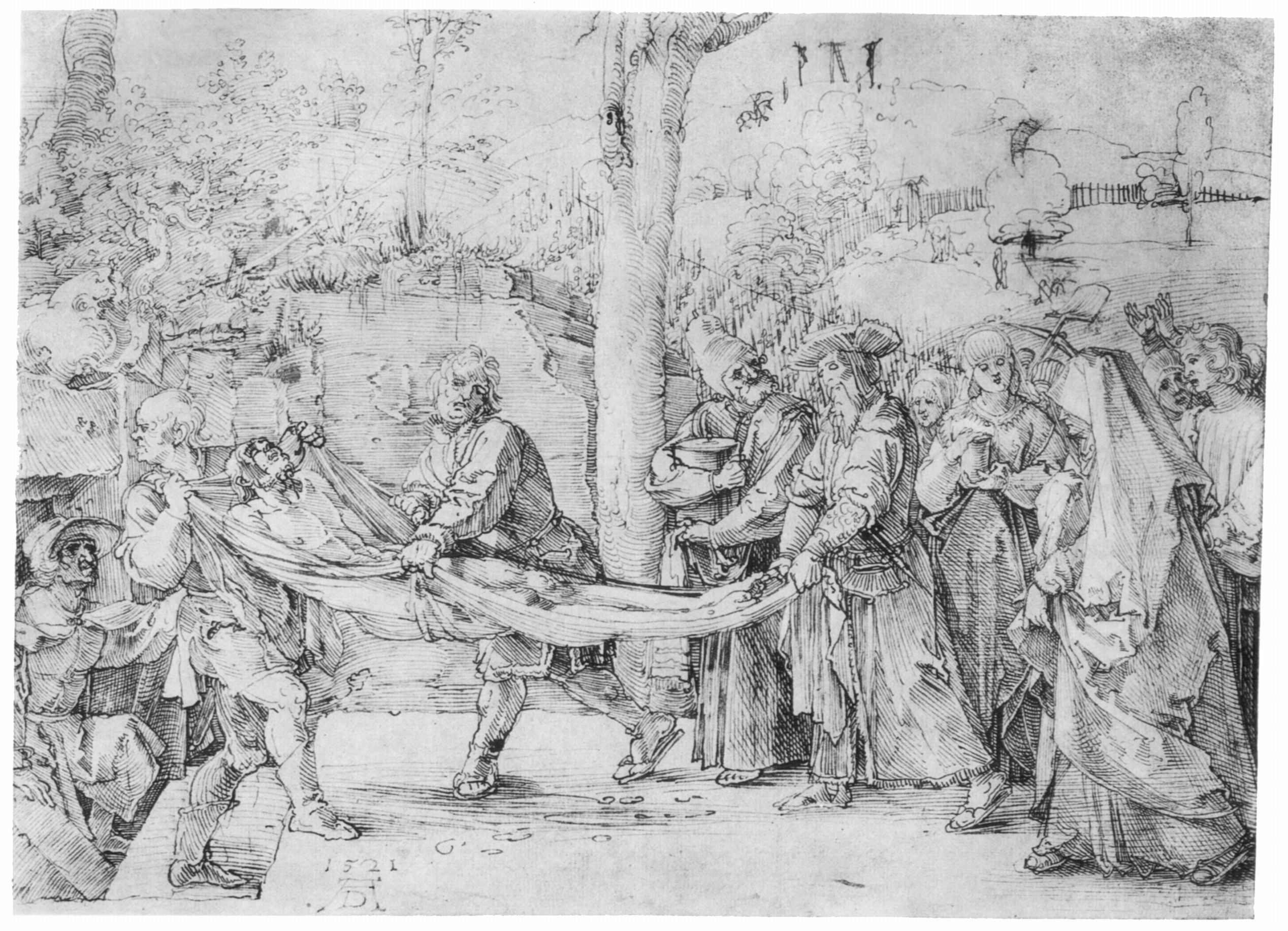The image is a detailed black-and-white sketch, possibly created with black ink, pencil, or charcoal. It portrays a historical or religious scene set outdoors, featuring a group of people dressed in period attire. The focal point is three men who are carrying a seemingly lifeless, naked man wrapped in a blanket, suggesting it might be a depiction of Jesus being taken down from the crucifixion. The man in the center grips the blanket firmly, while another supports the head, and a third, wearing a hat, holds the part of the blanket around the feet. Surrounding them are women dressed in long robes and headscarves, some positioned on the right side of the image, with one raising her hands in the air. In the background, there are additional figures, including a man holding a book or container and another ascending stairs. The setting includes a central tree, a fence, and several other trees, suggesting a park-like or historical landscape. There is no text within the image to provide additional context.